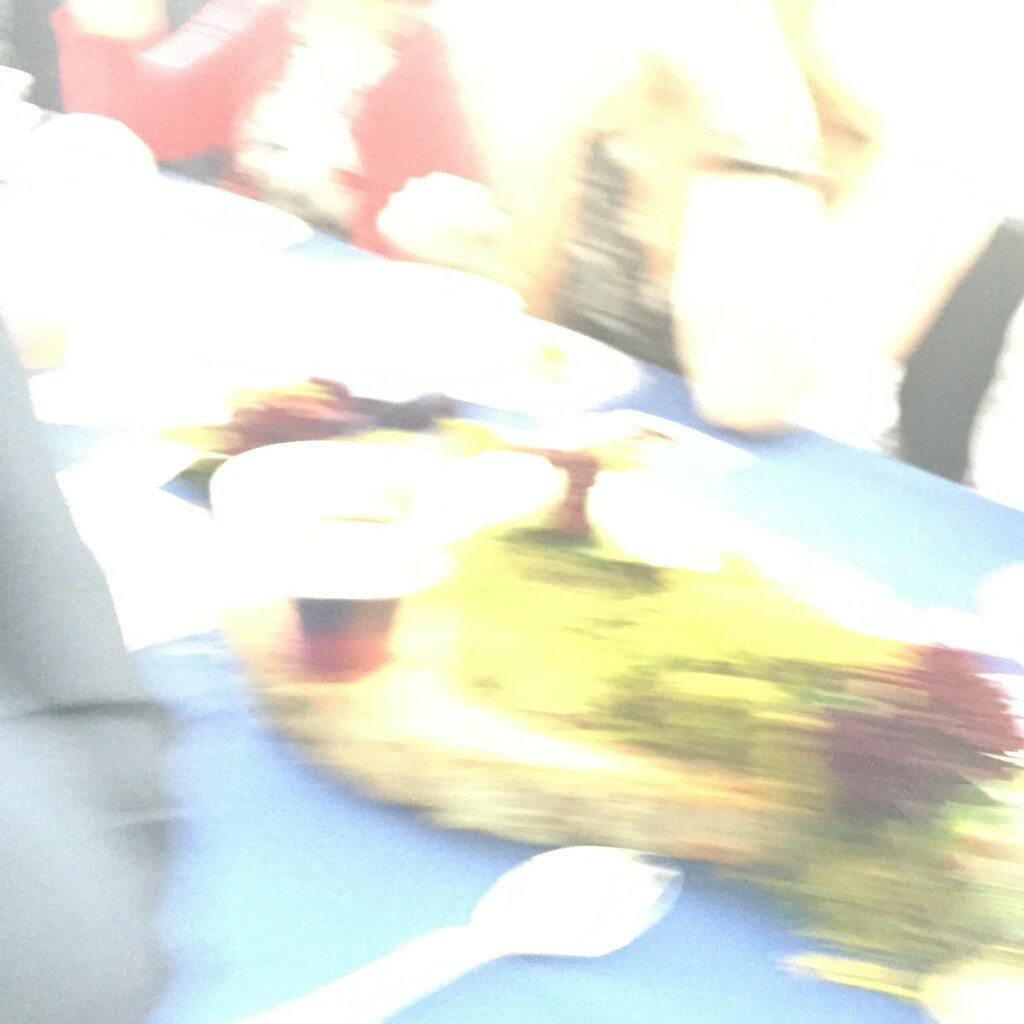A blurred image resembling a watercolor painting captures a dynamic scene, possibly distorted due to quick movement during the photo capture. Dominating the bottom center, a white shape with spoon-like contours is visible, immersed in light blue and dark purple hues to the left. Above this, a blend of beige, yellow, and dark pink adds complexity to the composition. The left upper section reveals dark pink, purple, and a faint, whitish circular shape, against a triangle of white layered with color splotches. A broader view suggests the frame showcases a blue tablecloth-covered table. Upon closer inspection, two figures appear to be seated at the table: one possibly portraying a woman with blonde hair and a dark jacket, and the other, a woman in a red jacket.